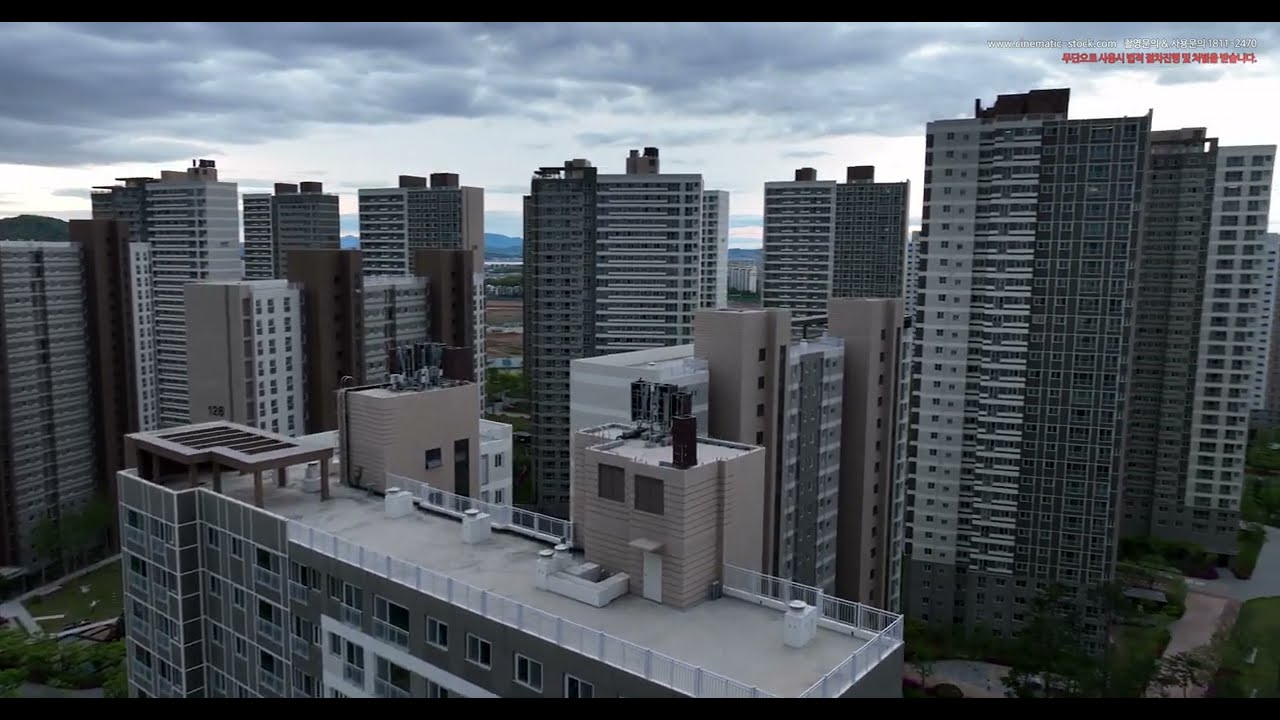This photograph captures a bustling cityscape, dominated by numerous tall buildings, likely apartment complexes, standing around 20 stories high. The skyline is punctuated by about seven white and gray buildings, each with flat rooftops hosting air conditioning units and utility sheds, lending a utilitarian aesthetic to the view. At the forefront of the image, a shorter, more square building stands out with its flat roof that appears accessible for walking. Surrounding this foreground building are walkways, patches of greenery, and bush-lined sidewalks on both the right and left sides, adding a touch of nature to the urban scene. The backdrop reveals a scenic mountain ridge beyond the towering structures. The overcast sky blankets the city in a muted, grayish hue, enhancing the overall somber and subdued ambiance of the day. There are no visible cars or people, further emphasizing the quiet, almost serene atmosphere amidst the urban sprawl.